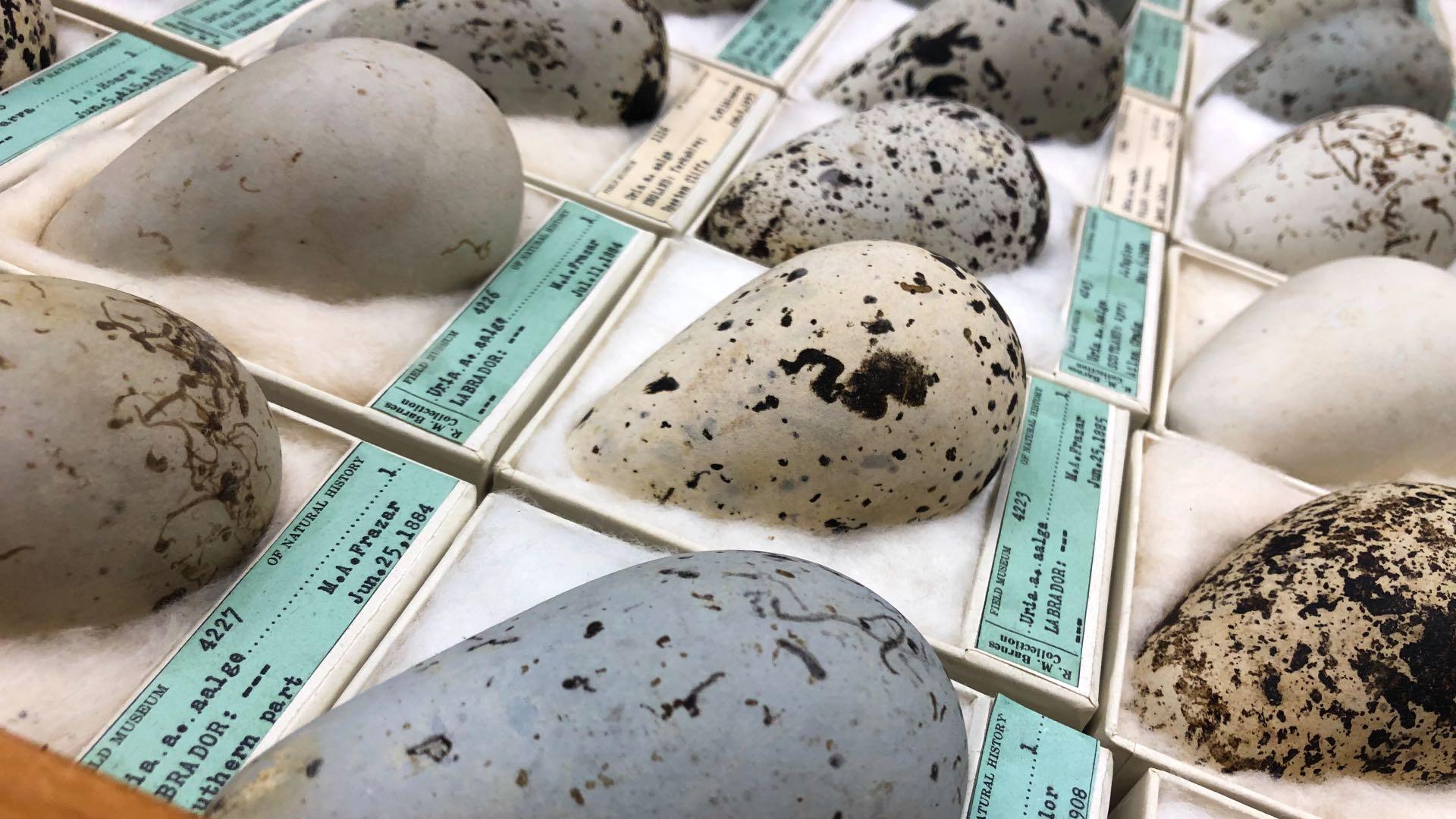The image portrays a display from the Field Museum of Natural History, showcasing egg-shaped objects that could either be eggs or stones due to the variability in their appearance. These artifacts are meticulously arranged in rows within individual white boxes that are lined with what appears to be white cotton or foam. The collection consists of four visible rows, each containing at least four to five objects. The eggs, or stones, exhibit a range of colors and patterns, including plain white, white with tan speckling, gray, gray with black speckling, tan with black speckling, and blue and black combinations. Each box has a blue label and indicates lot numbers such as 4227, 4228, 4226, and 4223, along with the name M.A. Frazar and a date of June 25th, 1884, suggesting the artifacts were discovered or cataloged on that date. The arrangement is illuminated by a predominantly amber-colored light source from the left side and likely supplemented by overhead lighting, enhancing the display's intricate details.